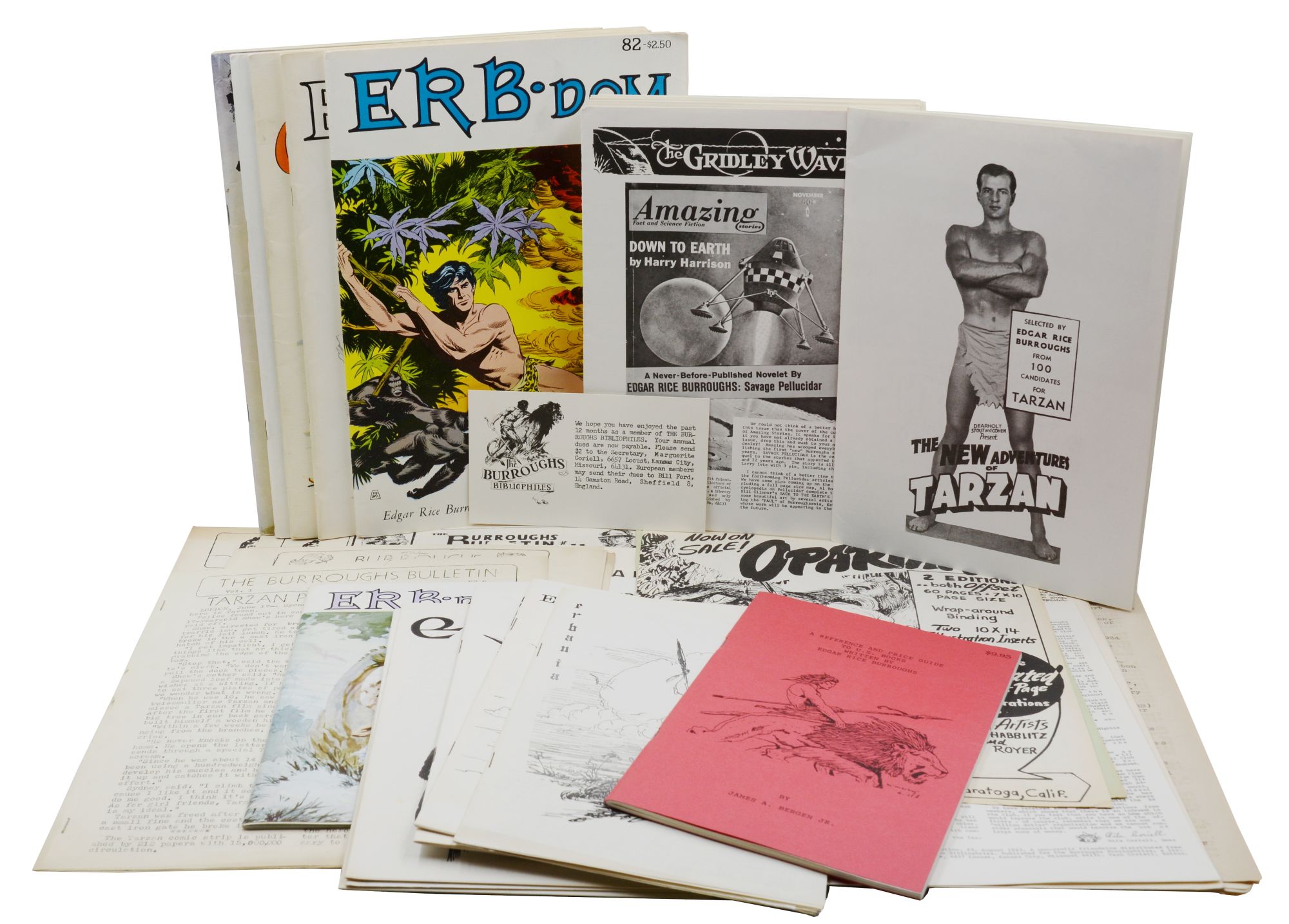The image depicts a collection of vintage magazines, books, and pamphlets with a central theme relating to Tarzan and the works of Edgar Rice Burroughs, all set against a white background. Dominating the right side is a black and white publication titled "The New Adventures of Tarzan," featuring a bare-chested man in a loincloth. Below this is a red pamphlet illustrating a prehistoric man with a spear riding or sailing a lion. In the center, a magazine titled "The Gridley Wave" showcases a never-before-published novelette by Harry Harrison, accompanied by an image of a planet and a rocket-like spaceship. Further to the left is another publication, "ERB-DOM" (issue number 82), with a blue and yellow cover depicting a cartoonish Tarzan amidst vegetation. Scattered throughout are black and white postcards and clippings, including an unreadable pink pamphlet. Some additional materials appear below these highlighted items, partially obscured but contributing to a rich collage of nostalgic and literary artifacts celebrating the legacy of Edgar Rice Burroughs.